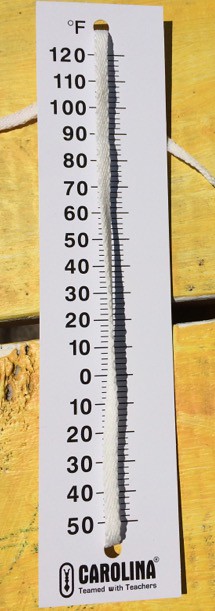The image features a white thermometer with black lettering and black graduations. It measures temperatures ranging from 120°F to -50°F. The thermometer is mounted against a pale yellow background with a distinct black stripe running horizontally across the middle, suggesting it might be an exterior wall. The thermometer bears a logo for the state of Carolina and an inscription indicating a partnership with teachers. Additionally, there is an enigmatic emblem inside an oval cartouche, resembling a 'Y' shape with a blob at its base, though the precise details remain unclear.